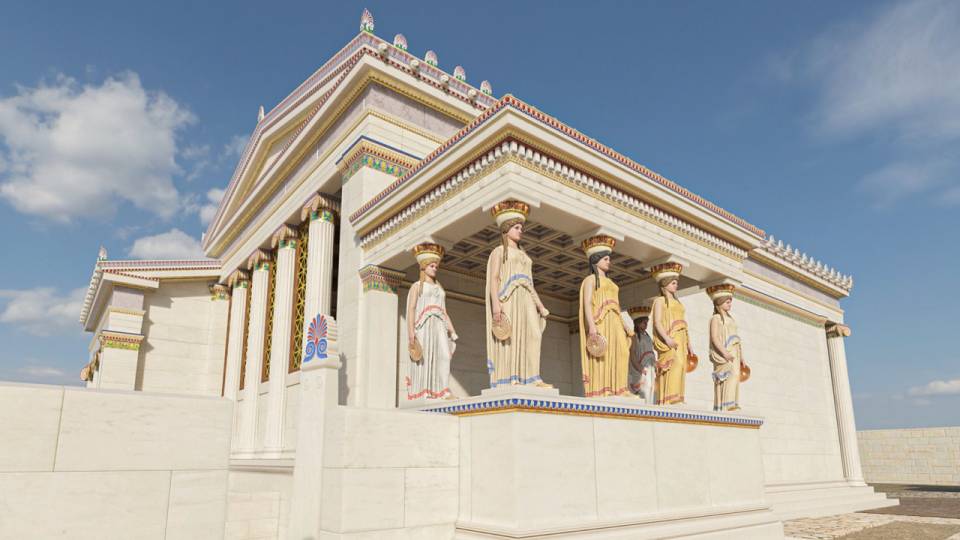The image depicts an elegant, ancient marble temple beneath a clear blue sky with minimal clouds. The structure is predominantly white, featuring intricate and elaborate carvings. The temple's architecture includes a row of five statues of women dressed in flowing gowns—one in white, one in cream, two in yellow, and another in white—standing between the base and the roof, effectively acting as supportive pillars. Notably, these statues appear to wear Egyptian-style crowns, contributing to the belief that the building might be of Egyptian origin.

Adjacent to the statues, there are additional pillars, with occasional gold accents adding to the temple's grandeur. The left side of the building reveals an L-shaped structure with a staircase leading up to the entrance. In the distance, the environment is arid, characterized by sand and further highlighting the vibrant blue sky. Also of interest, a colorful element resembling a peacock's tail, displaying blues and pinks, appears near the front of the temple, adding a touch of mystique to the scene.